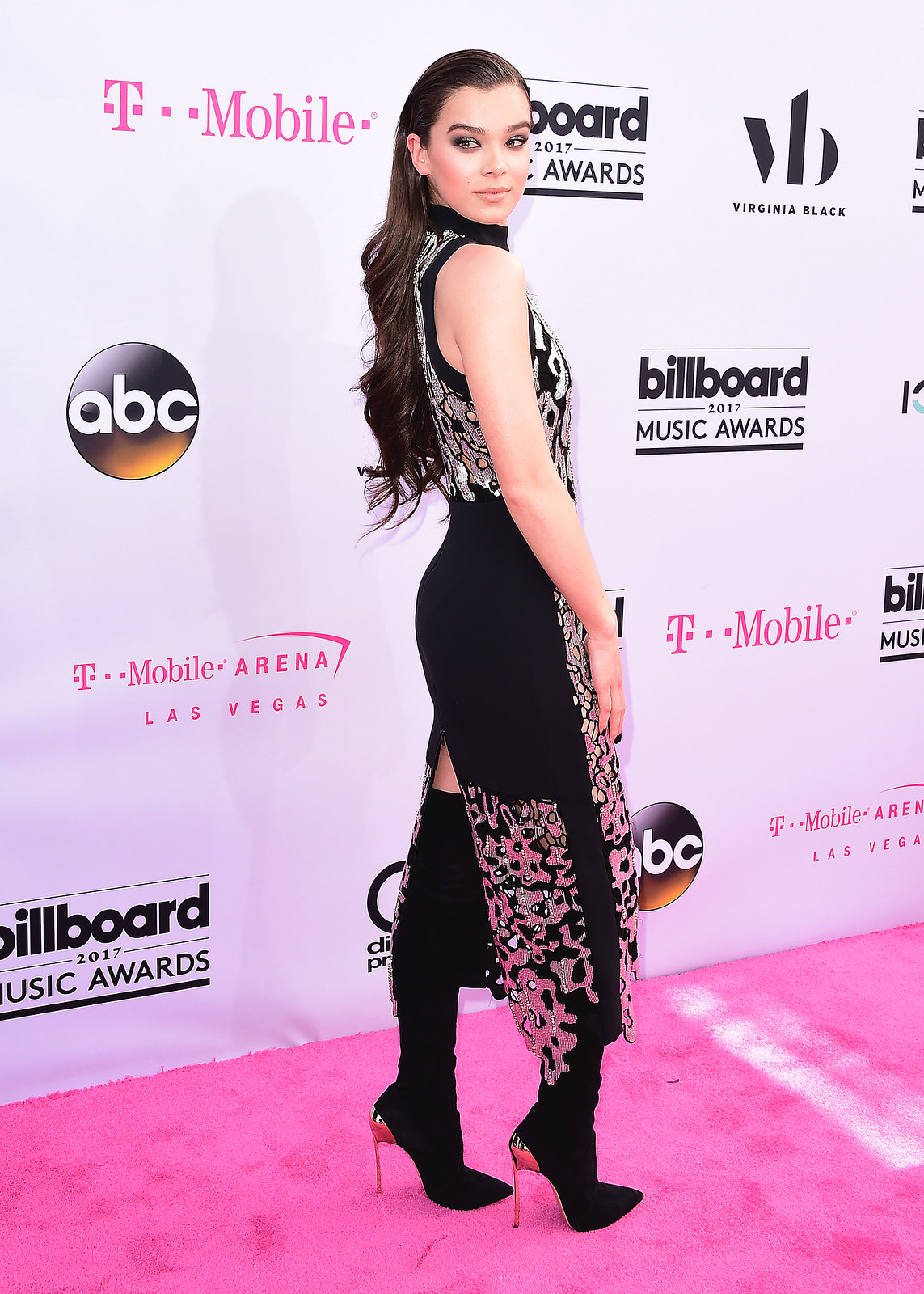In this elaborately detailed portrait-style photograph taken at the 2017 Billboard Music Awards, the young actress and musician Hailee Steinfeld is captured in a full-length body shot. Steinfeld, known for her role in "Hawkeye," is posing on a pink carpet awash with bright lights typical of these events. She has long, dark brown hair that cascades to the middle of her back, meticulously combed and styled. Her makeup gleams with a sleek, metallic finish.

Draped in an elegant black dress adorned with intricate pink and silver patterns, sequins, and gems, she exudes sophistication. Complementing her ensemble are striking black stiletto heels featuring gold spikes. Steinfeld is poised with expertise, glancing over her right shoulder just slightly off-camera, adding a touch of mystique to her demeanor.

The backdrop against which she stands is predominantly white, showcasing logos from the Billboard Music Awards, ABC, Virginia Black, T-Mobile, and the T-Mobile Arena in Las Vegas. The text "Billboard 2017 Music Awards" is prominently displayed, while the entire scene captures the quintessential glamour of a red carpet event, albeit on a pink carpet.